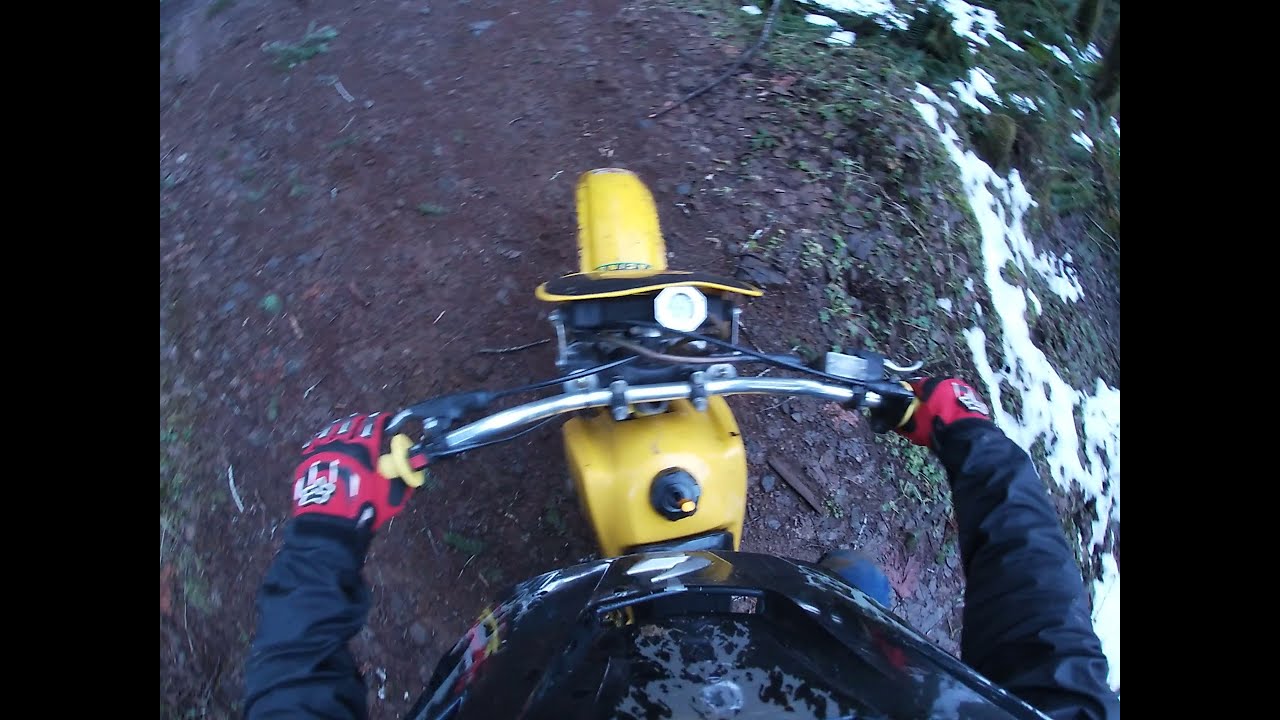In this image, captured from a GoPro-style point of view, we're riding along a compacted dark brown dirt path on a yellow motorcycle equipped with silver handlebars and yellow hand grips. The rider is wearing distinct red and black Fox Racing gloves, a black jacket, and a black helmet with a reflective visor. Below, the dirt trail is sprinkled with twigs, rocks, and some leaves at the edges, flanked by a variety of green vegetation. On the right side, small piles of melting snow are scattered near a steep drop-off, and a dark brown tree trunk is visible at the top right corner. Black brake cables and a handbrake are prominently seen, adding to the detailed view of the motorcycle gear. The overall scene captures the rugged terrain and the rider's careful navigation through this mix of dirt path and snowy landscape.